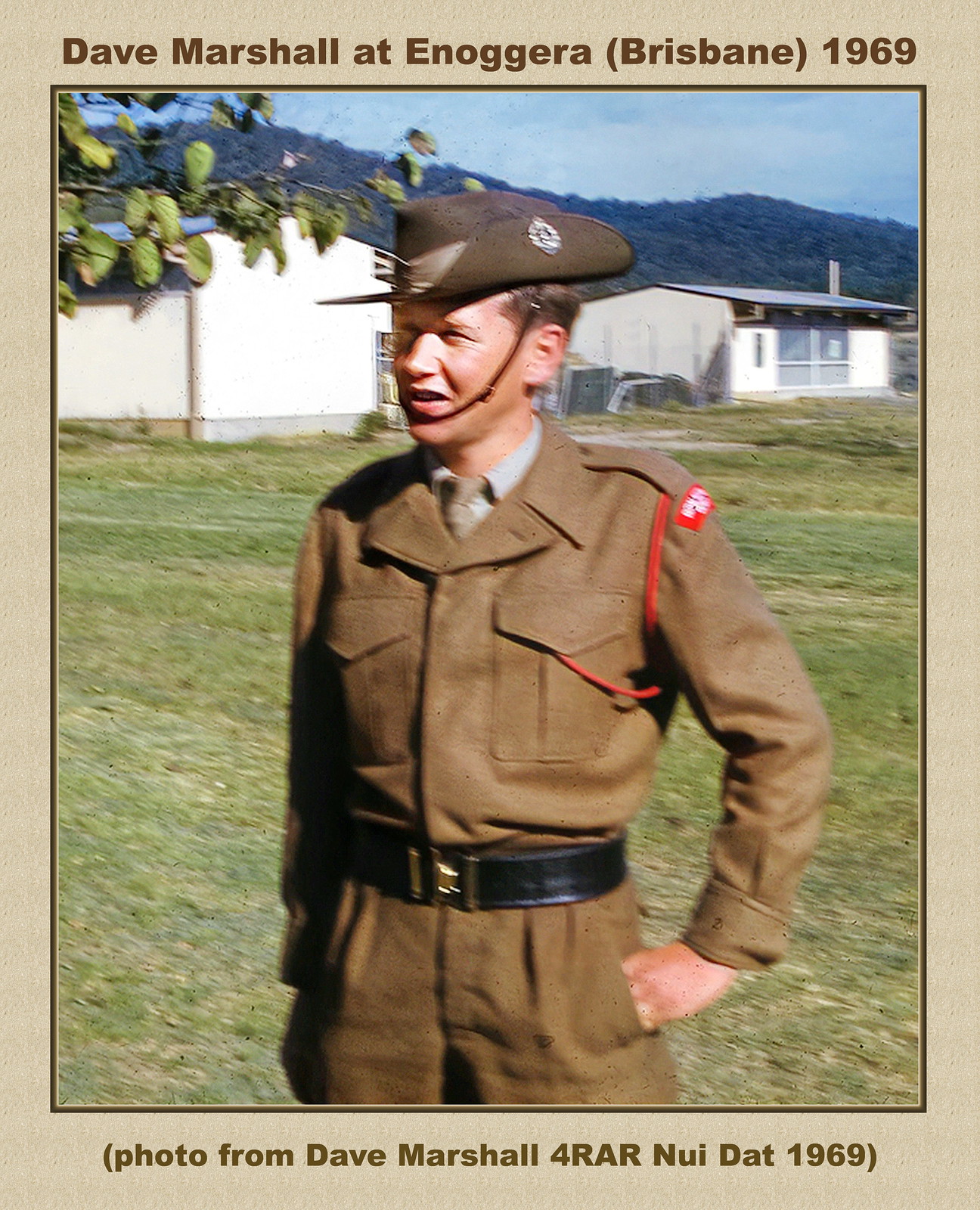The image captures a vintage photograph set within a beige matte border. At the top of the border, the inscription reads, "Dave Marshall at Enoguera, Brisbane, 1969," while the bottom of the border states, "Photo from Dave Marshall, 4 RAR, Noydat, 1969." Central to the photograph is a soldier, Dave Marshall, attired in a brown uniform complemented by a distinctive brimmed hat that curls up on one side and features a red badge on the left shoulder. He is standing in a grassy field, looking slightly to his left in a candid, unposed manner. Surrounding him, the backdrop includes white buildings and distant rolling hills covered in greenery, under a clear blue sky with scattered white clouds. The upper left corner of the frame also shows part of a tree branch with leaves. The overall scene suggests a bright outdoor setting, likely mid-day, situated in Brisbane.